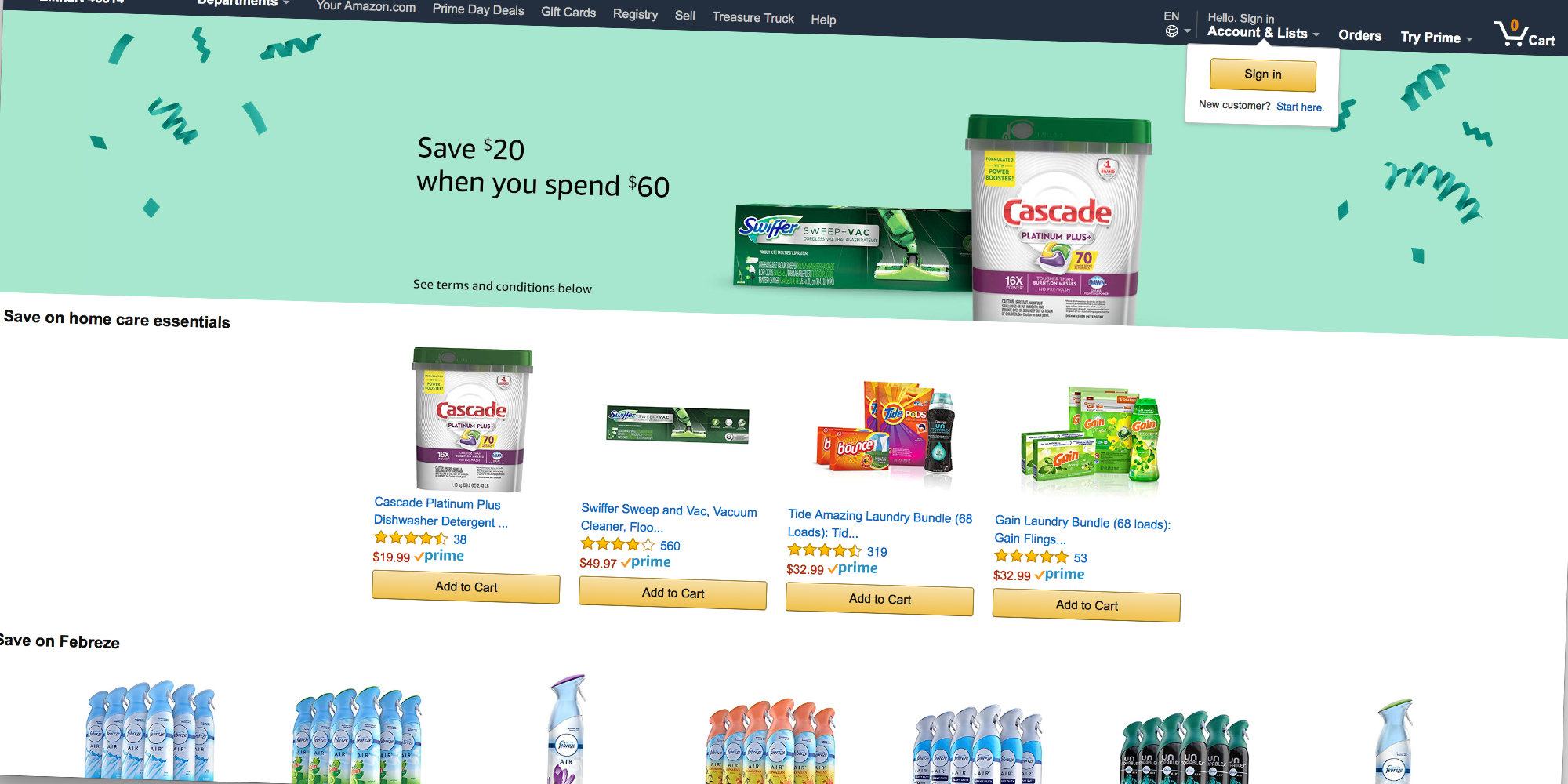This image is a tilted screenshot of an Amazon web page. The top gray banner appears angled to the right, causing the Account & Lists, Orders, and Try Prime buttons to skew, along with the shopping cart and sign-in icons positioned at the top right. A light green banner adorned with green confetti occupies the upper section, featuring images of Swiffer and Cascade products. To the left, it advertises "Save $20 when you spend $60." Below this banner, there is a "Save on Home Care Essentials" section displaying four horizontally aligned items: Cascade, Swiffer, a Tide and Gain bundle. Each item showcases yellow star ratings and red prices, accompanied by a Prime checkmark. Featuring prominently below and partially off-page are grouped varieties of Febreze air fresheners, labeled with "Save on Febreze" to the left.